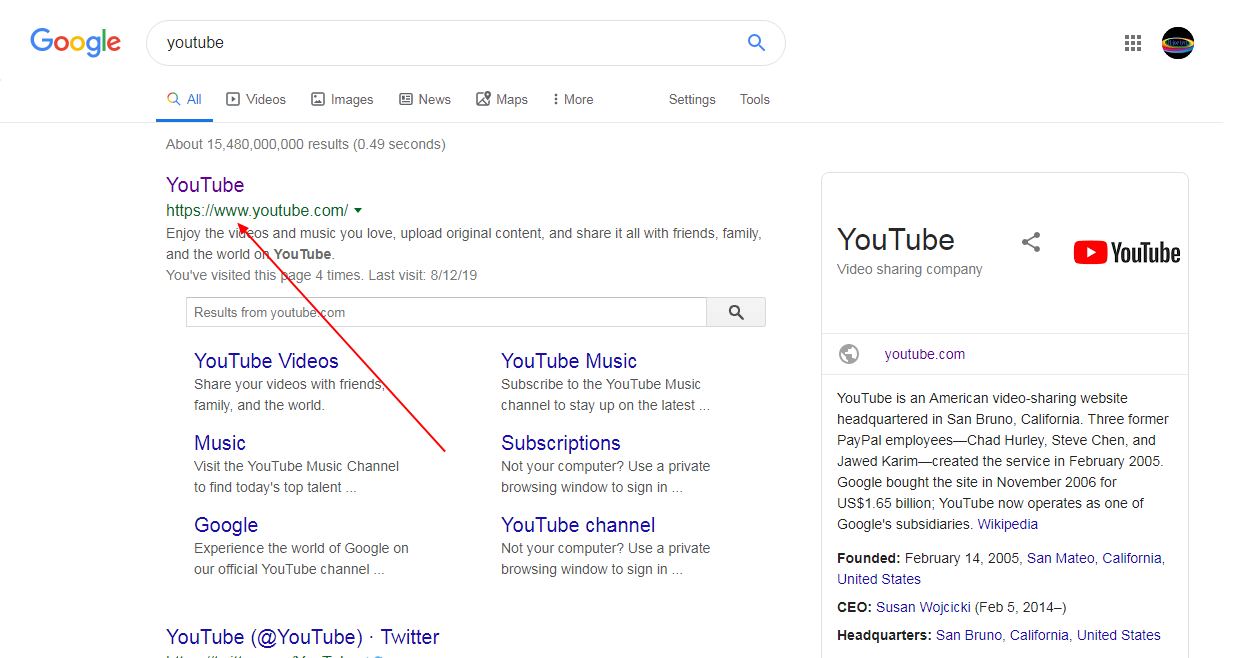In this image, a screenshot captures a desktop screen displaying the Google homepage. At the top left of the page is the iconic Google logo in its characteristic blue, red, yellow, and green colors. To the right of the logo is a prominent search bar showing the term “YouTube” typed in black text.

Above the search results are various filtering options, including "All," "Videos," "Images," "News," "Maps," "More," "Settings," and "Tools." The "All" option is highlighted in blue text with a blue underline, while the other options are displayed in grey.

Beneath the search bar, Google displays the number of results found for “YouTube” and the time it took to generate these results, written in grey text. The first search result is a purple hyperlink to YouTube, followed by the website URL in green text. A red arrow points to this link, emphasizing its importance.

On the right-hand side of the screen, there is an informational panel summarizing details about YouTube, such as its history, ownership, and founding date. This panel provides a concise overview of the platform, enhancing the user’s understanding of the search term.